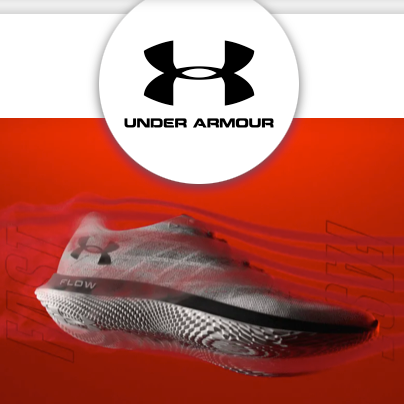This image, part of an Under Armour advertisement, features a clean, modern design. At the top of the image, a long, slender horizontal gray rectangle serves as a minimalist header. Directly beneath this header, a circular emblem showcases the Under Armour brand name, accompanied by the company's iconic logo—a stylized "U" that curves upwards meeting a mirrored "U" curving downwards, both rendered in black.

Centered below the logo, a vibrant red rectangle draws attention to a sleek Under Armour tennis shoe. This shoe, prominently displayed, is highlighted by lines cascading over it as part of the ad's dynamic artwork. The shoe itself is primarily a gray hue and is identified as the "Flow" model by the black line inscribed with the word "Flow," running along the upper part of the sole. The Under Armour logo is also visible on the heel of the shoe.

Enhancing the visual appeal, the word "FAST" is highlighted in bold red print in two instances: one vertically ascending on the left side and the other vertically descending on the right, emphasizing the shoe's emphasis on speed and agility.